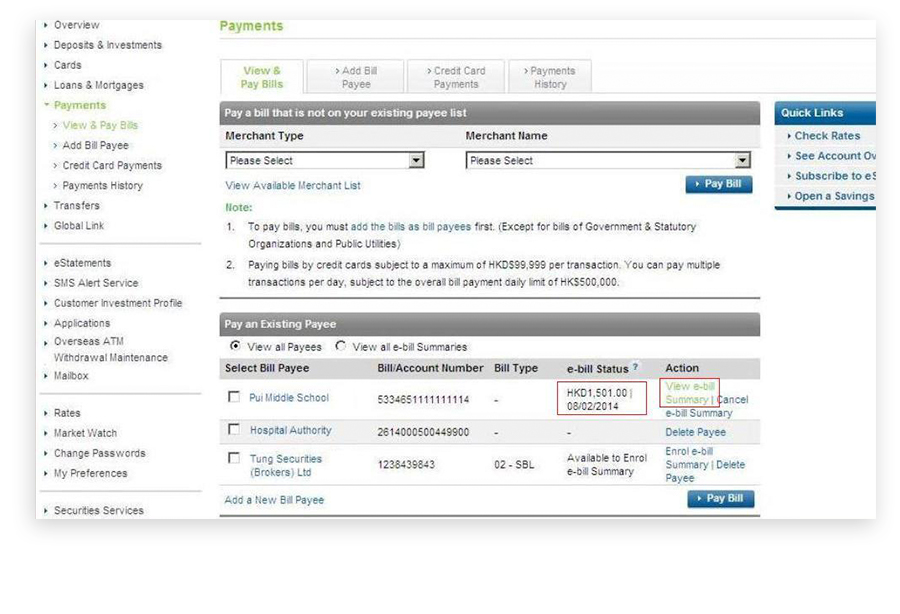The image depicts an online banking dashboard for Ansible Investments. The left side features a pane with a white and black background. The top section is titled "Overview" and displays various categories such as "Deposits," "Loans," and "Mortgages."

In green text, it says "Payments," with options below including "View and Pay Bills," "Add Bill Payee," "Credit Card Payments," "Payment History," "Transfer," and "Global Link." Each section is separated by thin gray lines.

Further down, there are additional options: "E-Statements," "S and S Alert Service," "Customer Investment Profile," "Application," "Overseas ATM," "Withdraw Maintenance," "Mailbox," "Rates," "Market Watch," "Change Passwords," and "My Preferences." Lastly, it includes "Security Services."

On the right side, at the top of the pane, "Payments" is highlighted in green. Below that, separated by a thin gray line, are several tabs: the first tab is white, labeled "View and Pay Bills" in green, while the following three are gray with darker text, labeled "Add Bill Payee," "Credit Card Payments," and "Payment History."

A white area with a darker gray border follows, containing text that says, "Pay a bill that is not on your existing payee list."

On the left, another section in blue titled "Quick Links" offers options like "Check Rates," "See Account," "Subscribe To," and "Open Savings." Adjacent to this, under "Merchant Type," it prompts to "Please Select" with an option to "View Available Merchant Lists." The layout is systematically organized for easy navigation.